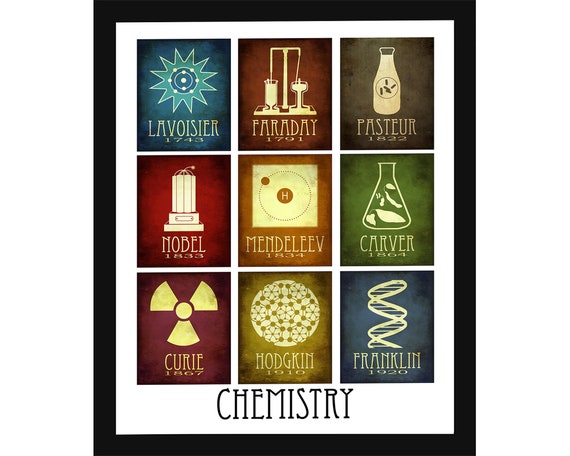The image is a framed poster titled "Chemistry" in black text at the bottom, set within a black frame and a white mat. Within the white border, the poster features the names and dates of nine prominent chemists along with multicolored artwork depicting their significant discoveries and accomplishments. Each section is uniquely colored, with hues of blue, green, red, brown, gray, orange, dark green, and dark purple enhancing the visual diversity. Starting from the top left corner, there is a blue image with a sunburst pattern labeled "Lavoisier" and dated 1743. Continuing, we have a depiction for "Faraday" dated 1791, characterized by two glass containers on a rectangular plate. To the right, "Pasteur" is listed with the date 1822 next to a sealed bottle with rods. Other featured chemists include "Nobel" (1833), "Mendeleev" (1834), "Carver" (1864), and "Hodgkin" (1910). Notably, "Curie" is highlighted against a red background with a radiation symbol, dated 1867, and "Franklin" is listed as 1920. The entire composition is a vibrant array of colors and symbols, each section celebrating the trailblazing achievements in the field of chemistry.